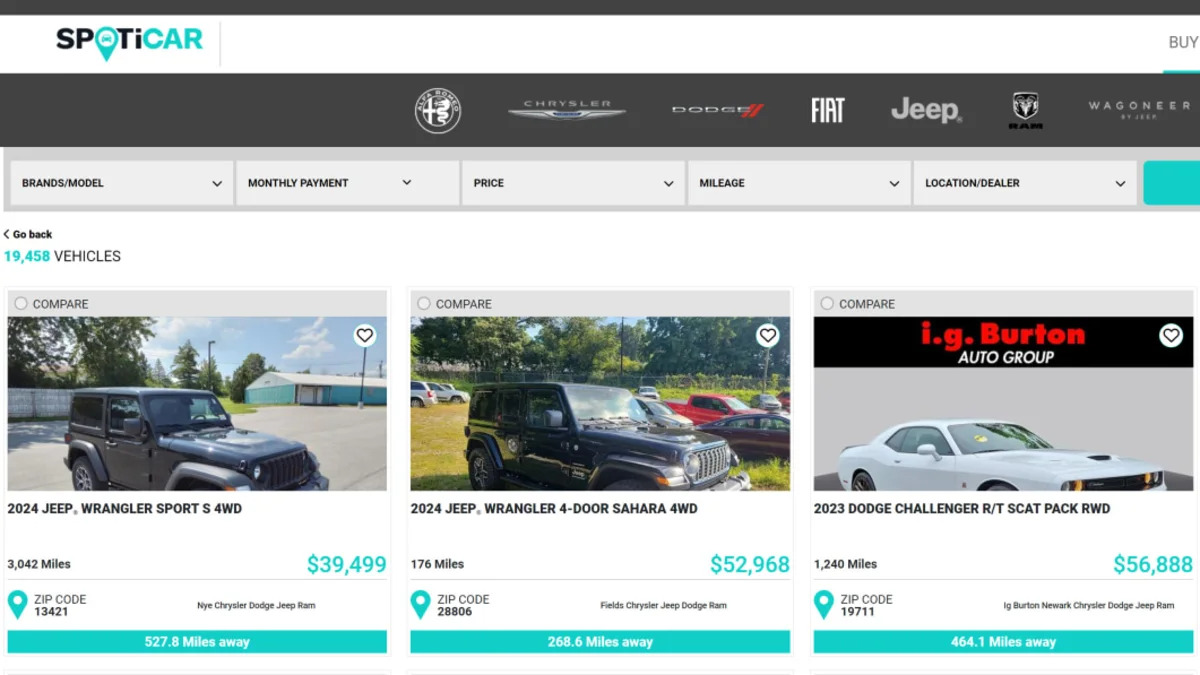This image depicts a structured and detail-rich layout of a car dealership website interface. 

At the very top, a black bar spans the width of the page, immediately followed by a white bar below it. On the left side of the white bar, the brand name "SPOTACAR" is prominently displayed with a stylized logo: an uppercase "S" and "P" in black, a blue "O" featuring a car icon, a black uppercase "T" followed by a lowercase "i," concluding with uppercase blue letters "C," "A," and "R." 

On the right side of the same white bar, the word "BUY" is highlighted with a blue underline signifying an active or selected state. Directly below, another black bar houses various car manufacturer logos, including notable names such as Chrysler, Dodge, Fiat, and Jeep.

Further down, a gray bar presents a series of drop-down menus for refined searches. These menus are labeled: "Brands," "Model," "Monthly Payment," "Price," "Mileage," and "Location/Dealer." Additionally, a small blue box sits to the right of these search filters.

Beneath this gray bar, the phrase "Go Back" appears alongside a display of "19,458 vehicles," indicating the total number of vehicles available for browsing. Below these figures, three vehicle listings are shown, each with a "Compare" checkbox option featuring an empty circle above it. 

The first vehicle listed is a "2024 Jeep Wrangler Sport S" with a four-wheel drive. The second is a "2024 Jeep Wrangler Four-Door Sahara," similarly equipped with four-wheel drive. The third listing features a "2023 Dodge Challenger R/T Scat Pack" with rear-wheel drive.

Overall, the interface is designed to make it easy for users to navigate car options and comparisons efficiently.